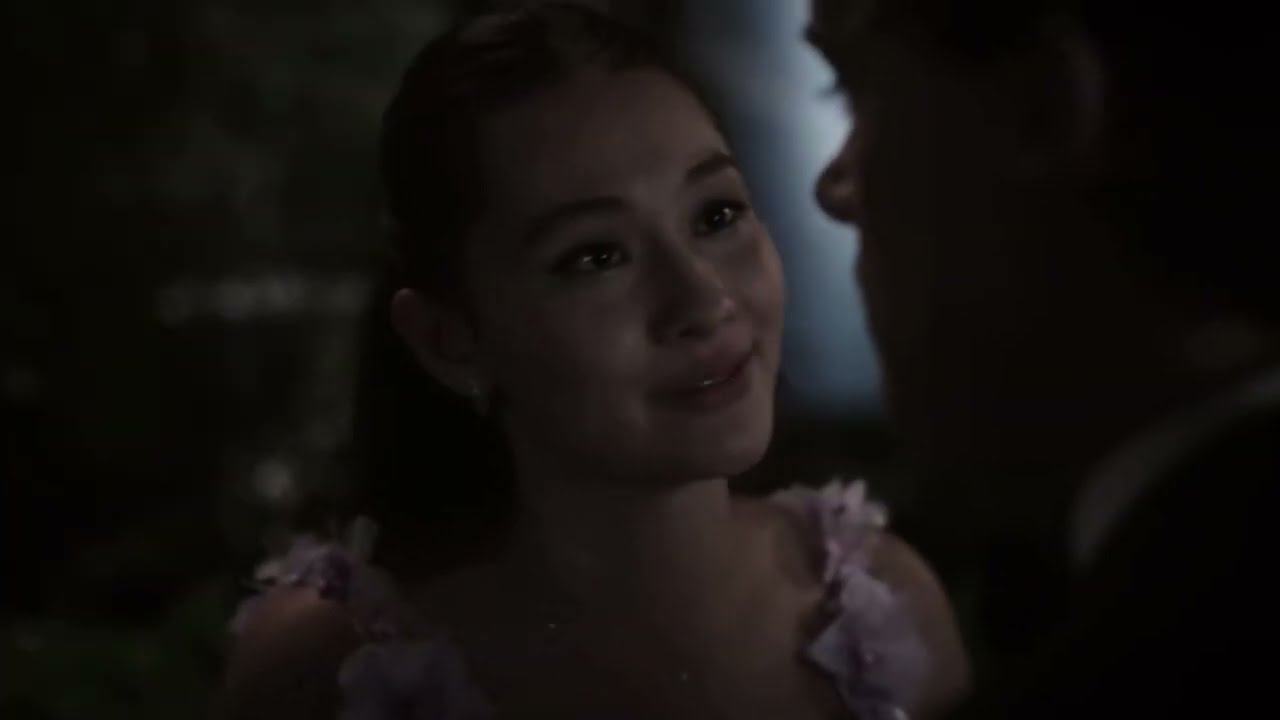The still image appears to be a frame from a movie scene, depicting a dimly lit, intimate moment between a young Asian woman and a man. The woman, who seems to be in her late 20s, has light skin, dark long hair draped down her back, and brown eyebrows. She wears red lipstick and a pink dress adorned with floral straps, possibly lavender or pink flowers. Her head is slightly tilted to the left, and she gazes lovingly and intently at the man, her mouth slightly upturned as if about to speak. The man, positioned on the right-hand side of the image, is partially visible, with only the side and back of his head, the outline of his nose, and his eyelashes discernible. He wears a black suit with a white shirt, appearing lighter-skinned. The image is somewhat fuzzy and dark, possibly suggesting an outdoor nighttime setting, with blurry colors in the background and a light source between their faces adding a soft glow to the scene.